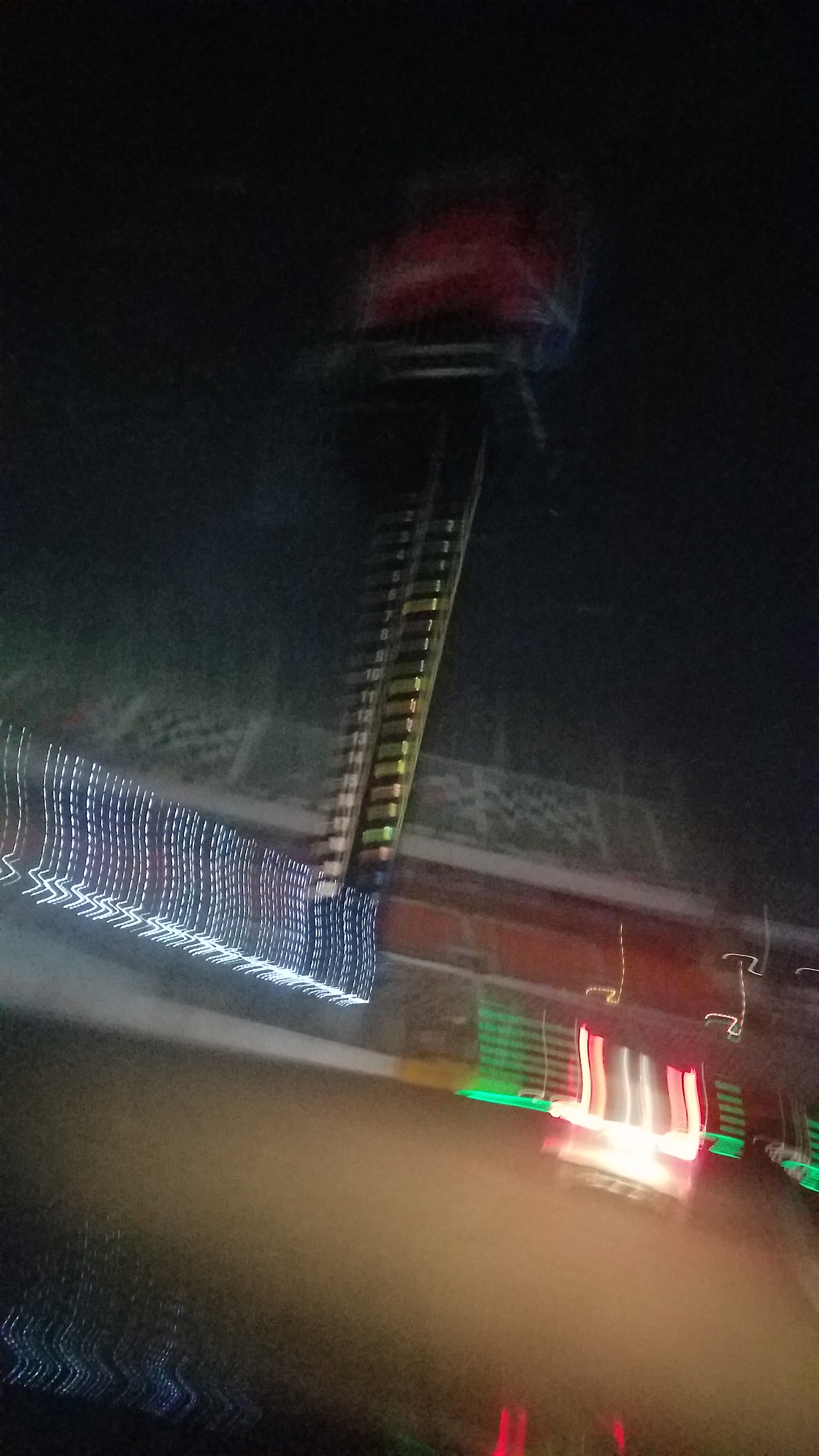A nighttime outdoor photo captures a blurry and dynamic scene at what seems to be a racetrack. In the distance, green and white spectator stands are visible, with rows of empty chairs looming beneath them. The foreground is dominated by a brown dirt track, and a black tower equipped with lights stands prominently on the left side of the image. The photo is characterized by numerous light streaks of varying colors—including red, white, blue, and neon green—adding a vivid, chaotic energy to the otherwise deserted venue. The absence of people accentuates the sense of motion and light, set against the static backdrop of empty stands and the quiet dirt track.